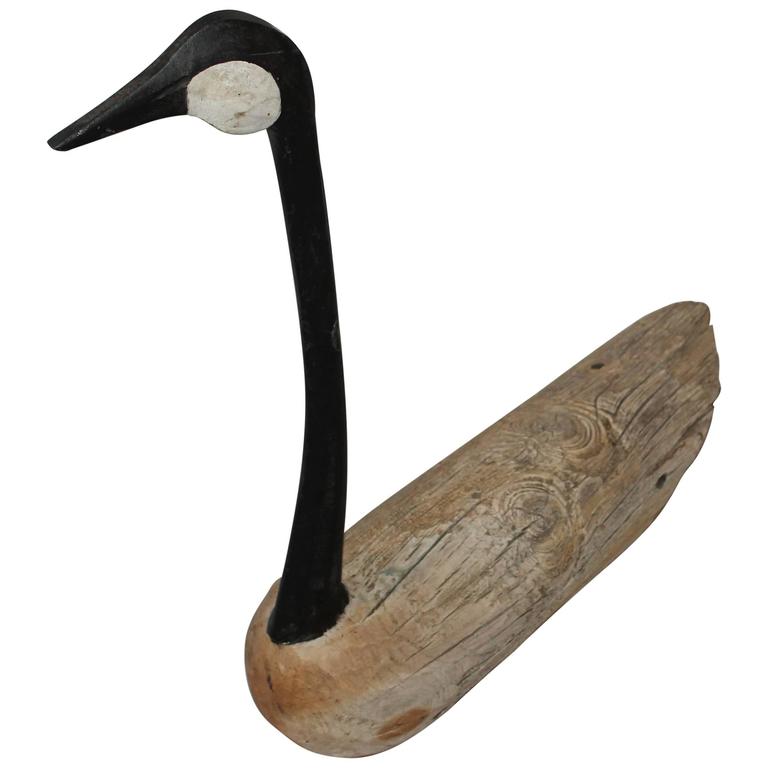This image is a close-up of a wooden sculpture depicting a waterfowl, possibly a swan or a duck. The piece is crafted from a rustic wooden log, which retains its natural imprints, patterns, and imperfections, including visible knots and small holes on the left and right sides. The lower section of the sculpture has been smoothed out but remains untreated and unpainted, preserving the wood's organic texture. Affixed to this base is the elongated neck of the bird, which is slender and gracefully arches upward, connecting to a detailed head.

The head and neck of the waterfowl are painted black with white accents on the cheeks, giving a stark contrast against the natural wood. The white paint forms a prominent circle on each side of the face. The beak is carefully shaped, tapering to a fine point, and appears almost metallic in finish, though it is crafted from wood. The back end of the wooden log is subtly frayed, adding to the appearance of feathers. The entire sculpture is set against a white backdrop, highlighting the intricate details and craftsmanship of the piece.